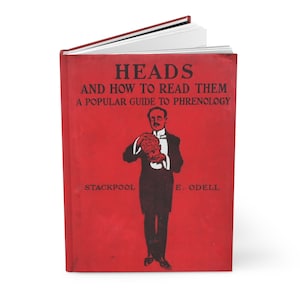The image features a small, hardback book standing up against a plain white background, open to reveal its white pages. The cover of the book is a solid dark red with bold black text. At the top, it reads "Heads," and beneath that, "and How to Read Them." Further down, it states, "A Popular Guide to Phrenology." At the center of the cover is a detailed drawing of a man with black hair and a black mustache. His face, along with his hands and the head he's holding, are painted in the same red as the book's cover. He is dressed in a black formal suit with a high-collared white shirt and black pants. His feet are positioned with the heels together and toes pointing outward. The drawing is flanked by the name "Stackpool E. Odell" in black text on either side of his waist.